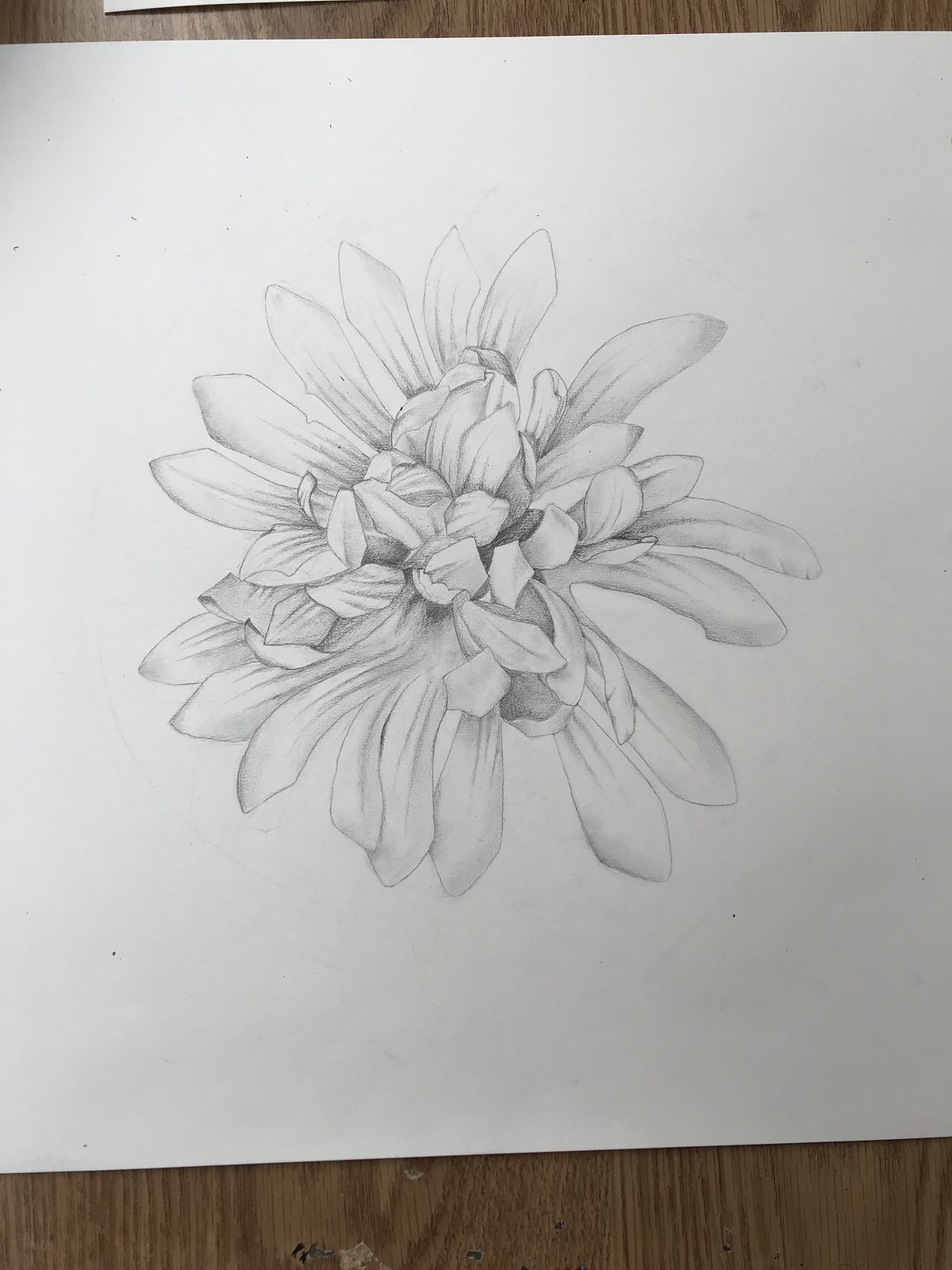This detailed pencil drawing showcases a partially-opened flower blossom, meticulously rendered on a sheet of paper that appears grayish in the photograph, contrasting with the medium brown wooden table it rests upon. The flower features an outer circle of approximately 15 to 20 delicately drawn petals, predominantly white with subtle shading towards their bases. These outer petals surround a more densely clustered center, where the petals seem to overlap and bend over each other, indicating that the bloom has not fully opened. The intricate layering of the inner petals conceals the stamen, carpel, and stigma, adding a touch of intrigue and anticipation to the drawing.